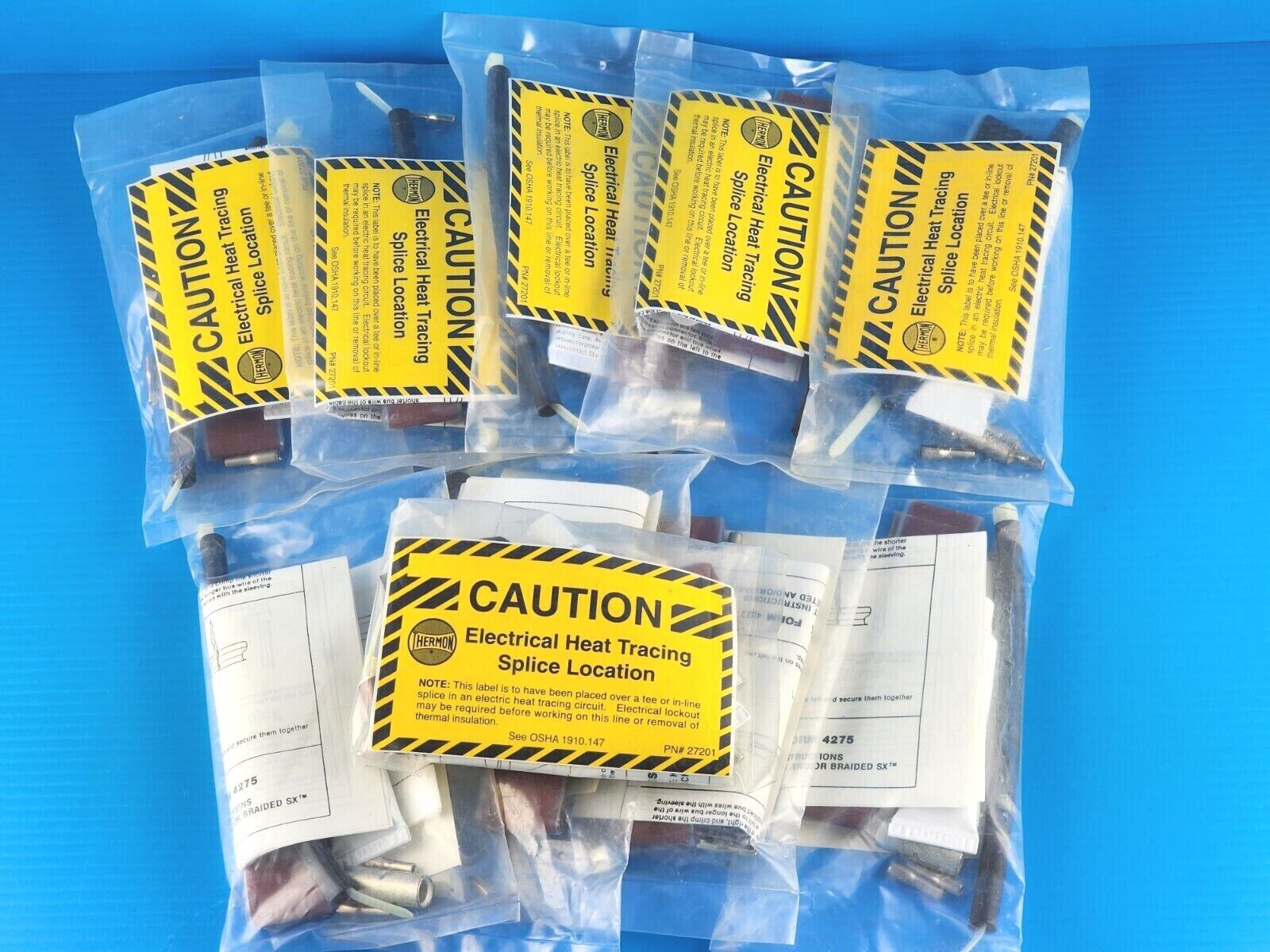This photograph features a neatly arranged collection of ten plastic packets situated against a blue backdrop, which appears to be the bottom panel of a box with a textured, lined design. The packets are identical and each contains a folded piece of white paper along with various elements. Prominently, each packet is marked with a yellow warning strip resembling hazard tape. At the center of this strip, set against a plain yellow background, is the text "CAUTION, ELECTRICAL HEAT TRACING SPLICE LOCATION" accompanied by a circular logo adjacent to the phrase. Beneath this warning, there is additional smaller text providing more detailed information. The image meticulously captures the organized presentation and detailed labeling typical of safety-related products.